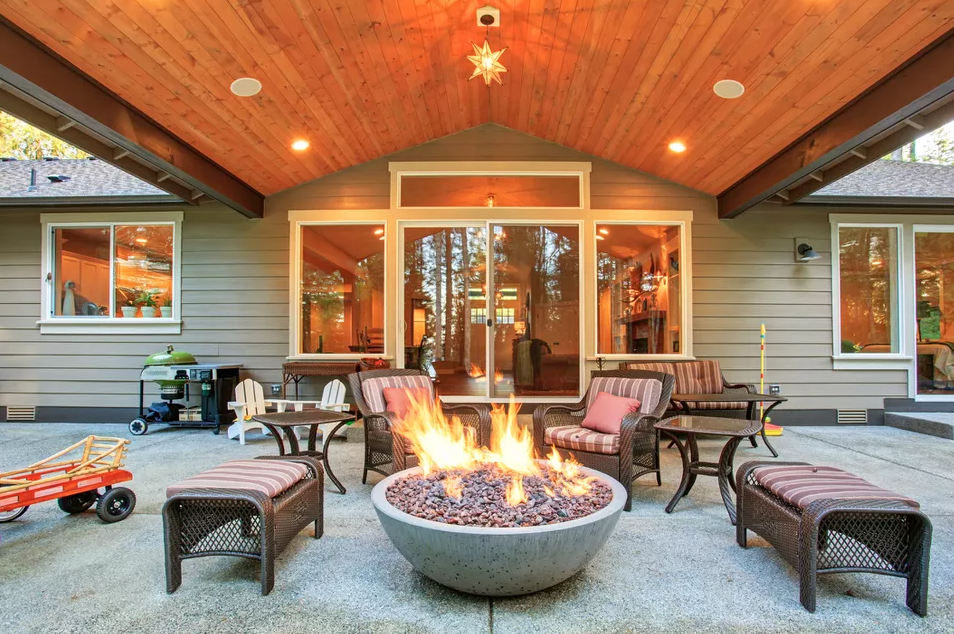The image depicts a cozy, well-equipped patio area at the back of a modest yet charming house. The patio is sheltered by a beautifully crafted wood ceiling with recessed slats, offering protection from the elements. Hanging from the ceiling is an eye-catching star-shaped light that resembles a Christmas tree topper, adding a whimsical touch to the space.

The seating arrangement includes two backless benches and a matching love seat, all with coordinated strap cushions. Additionally, there are wicker chairs with armrests and similarly cushioned seats, adorned with solid-colored throw pillows in shades of mauve or salmon. Accompanying the seating are two side tables that share the same design as the chairs and benches.

At the center of this gathering area is a large, stone fire pit, emitting lively flames, perfect for warmth and ambiance. Surrounding the fire pit are numerous seats, suggesting the hosts enjoy entertaining guests or have a large family. 

The patio overlooks the house through double glass doors, flanked by large windows, providing a clear view inside. Off to the sides, various outdoor items like a broom, a barbecue grill, a children's table and chairs, and a half-visible wagon add to the lived-in feel of the space.